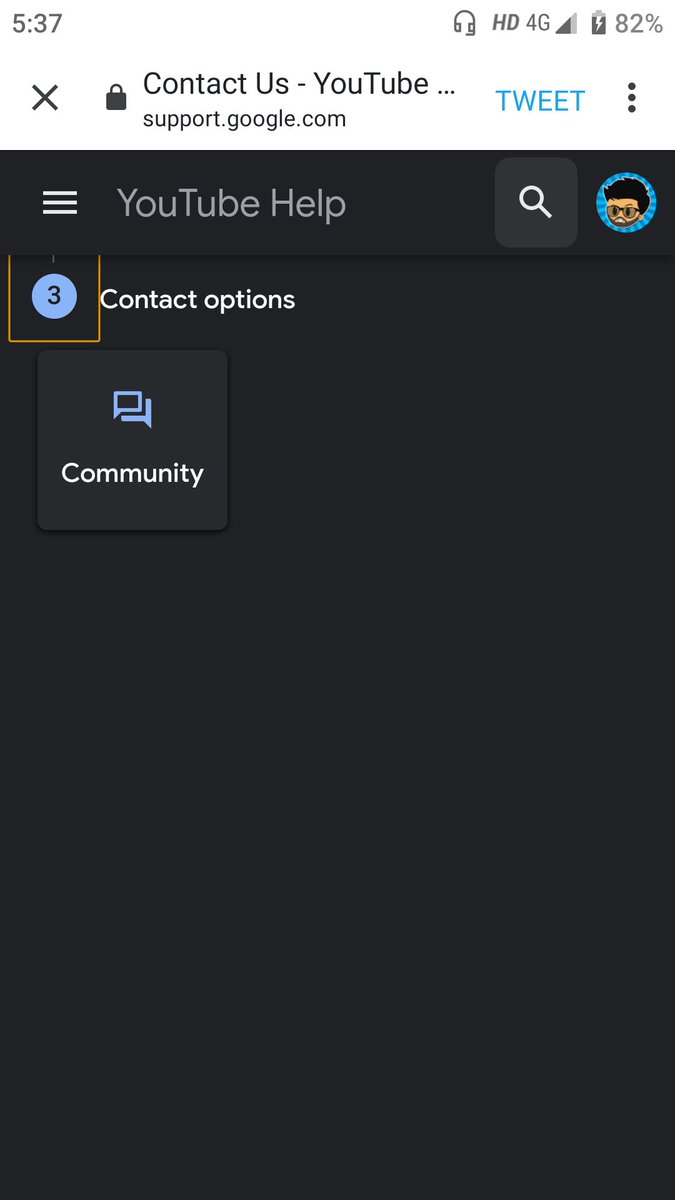Screenshot of a YouTube Support Page:
At the top of the page, there is an "X" icon, followed by a lock icon. Next to the lock icon, the URL reads "contactus-youtubesupport.google.com." To the right, in blue text, it says "Tweet," and further to the right, there are three vertical dots.

In the top left corner of the screen, the time is displayed as 5:37. The main section of the screenshot features a large black square with a black background. At the top of this square is a menu icon consisting of three white lines, and next to it, the text "YouTube Help" is shown. Adjacent to this, there is a search icon, followed by a circular icon displaying a cartoon male face.

Below this, there is a bordered square outlined in yellow with a black center. Inside the square is a blue circle containing the black number "3." Next to this, the text reads "Contact Options." 

Beneath this section, there is another black box with the word "Community" printed in white. Accompanying this text is a blue chat icon.